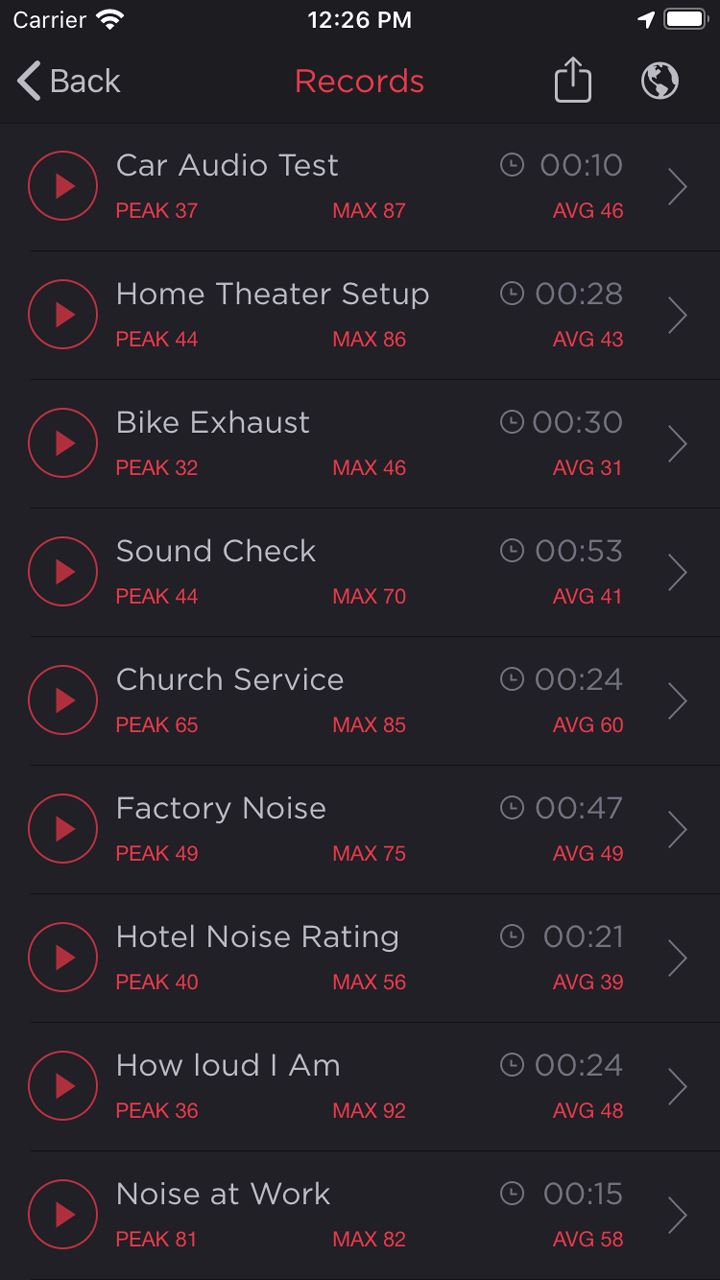This image is a detailed screenshot of a cell phone displaying a music or audio management application interface labeled "Records." The background is entirely black, creating a high contrast for the various on-screen elements. 

In the top left corner, the text "Carrier" is displayed in white, adjacent to a fully filled Wi-Fi icon. Centrally located at the top is the time "12:26." On the right side, there is a full battery icon with a small arrow pointing upwards and to the right, indicating charging or indicating directionality. Adjacent to "Carrier," there is a gray 'greater than' symbol pointing left, beside the word "Back" in gray text.

Dominating the center of the screen, the word "Records" is prominently written in red. To the right, a globe icon in gray and black signifies global options or settings. Next to it, there is a download icon outlined in gray with a black interior, featuring a gray arrow pointing upward.

Beneath the main header, a black circle with a red border houses a red play icon. To the right of this play button, white text indicates the type of audio listed as "Car Audio Test." Following this, a clock icon is displayed, showing a duration of "00:10 seconds." Further to the right, a red and gray 'greater than' symbol points right.

Underneath the "Car Audio Test" text, further audio specifics are listed: the terms "Peak" (37), and "Max" (87) are shown. Additionally, below this, "Avg" (46) in red records average levels, indicative of audio statistics.

Each audio entry follows a similar format, though the numbers differ for each category, providing specific audio metrics for each file listed.